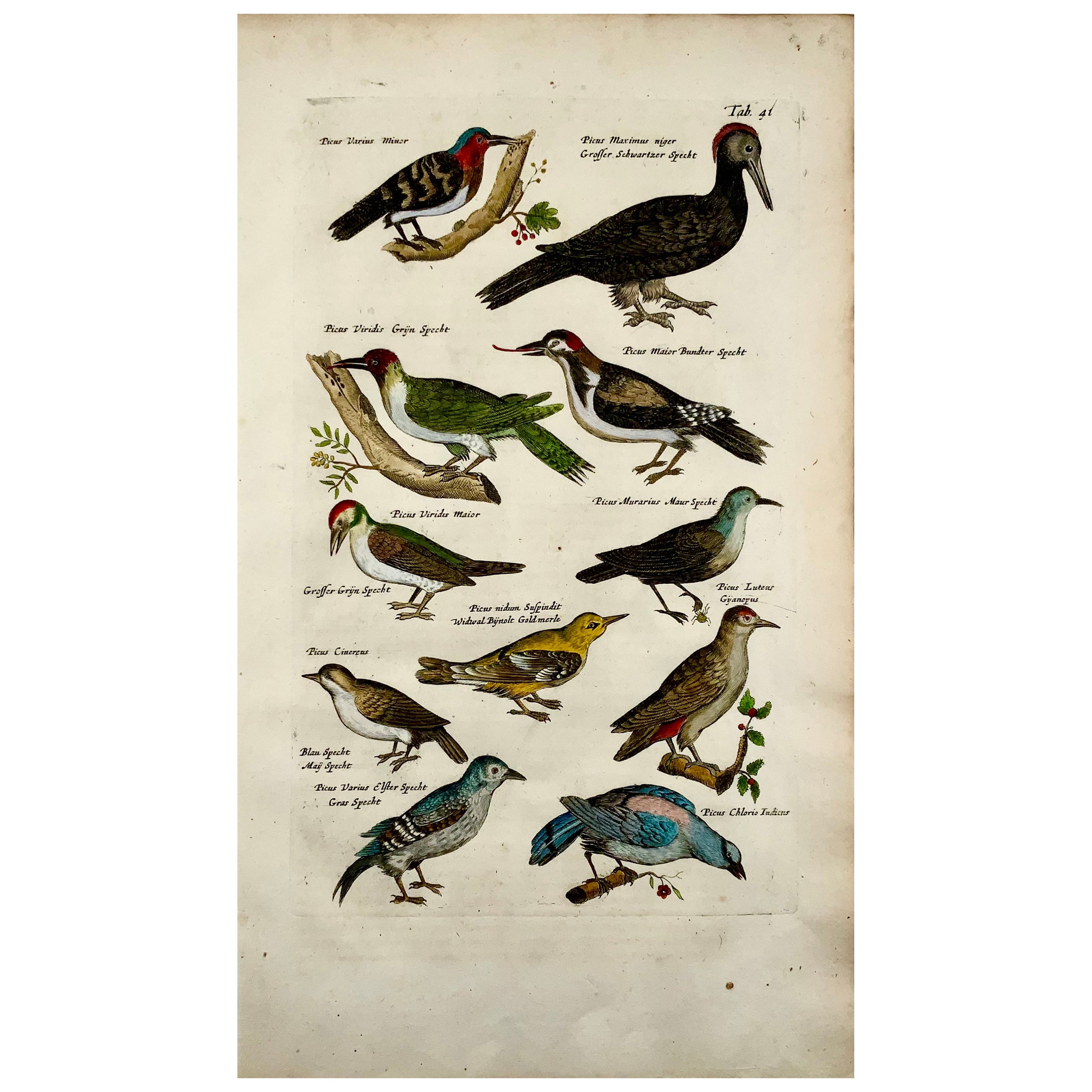The image showcases an ornithological illustration featuring 11 distinct species of birds, meticulously drawn on aged, grayish-tan parchment paper. At the very top, a bird with a green and red head, brown chest, and black wings pecks at a branch with its long beak. To its right stands a bird with a slightly lighter-colored head accentuated by a striking red mohawk, black body, light gray eye area, and a long gray beak. Below these top birds, nine others are depicted in vibrant shades of greens, yellows, blues, and reds. 

Among them, a green bird with a white belly and red head, a vividly yellow goldfinch, and another bird with a red head, white belly, and a peculiar long red tongue. Nearby, a small bird dons a green and red head, a white belly, and brown wings. A bird with a bluish-green head and curved beak, brown belly and wings, and a white chest stands prominently. Several birds below have unique colorations: from blue birds with combinations of green, gray, and brown, to a bird with pink on its back and predominantly blue plumage.

Handwritten labels in small print accompany each bird, though the text is slightly hard to read, suggesting this illustration might have been part of an old, weathered textbook intended for documenting various bird species.